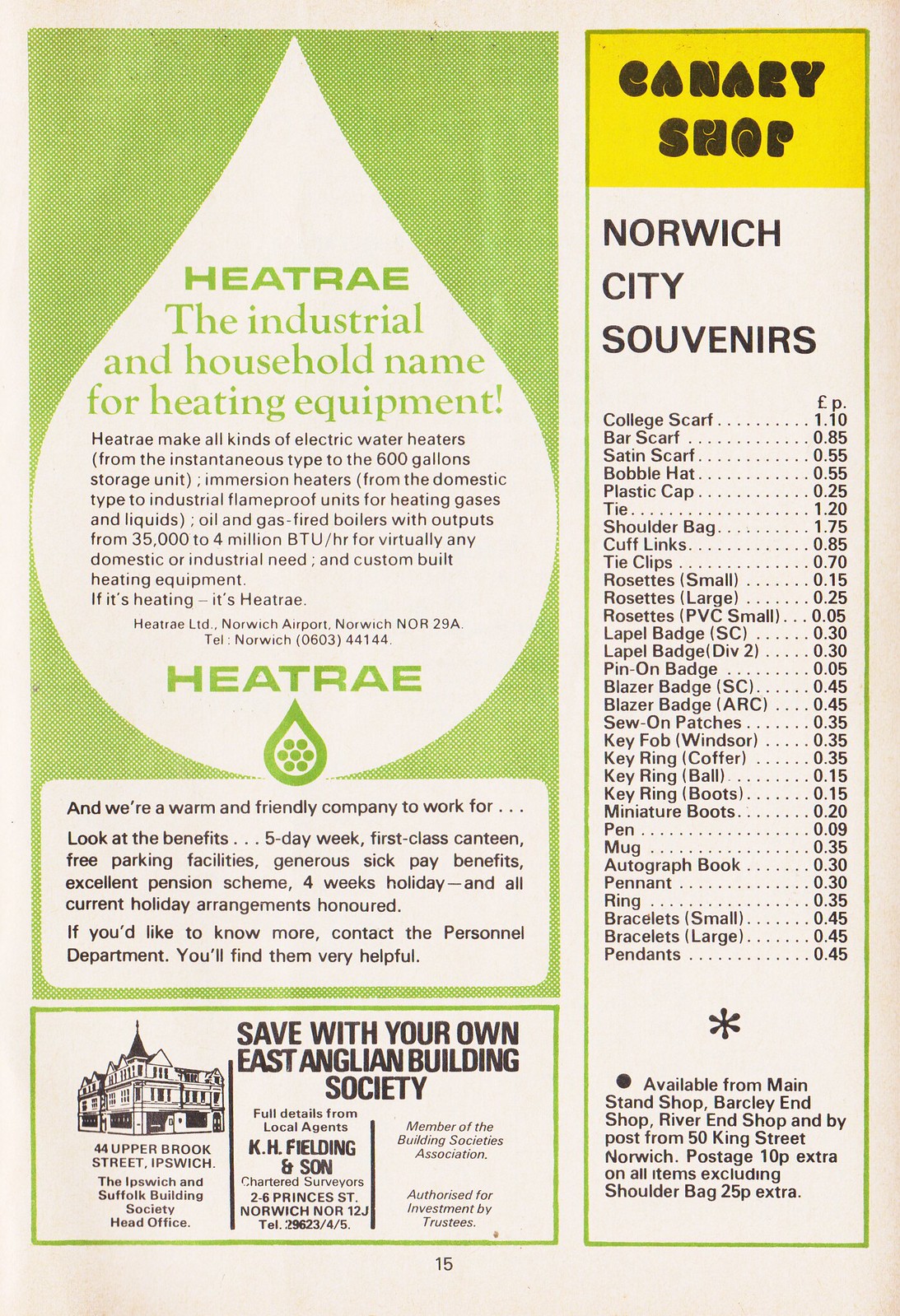The image features a black-and-white page from a historical soccer program, accented with green and yellow highlights. Predominantly, the top right section showcases the "Canary Shop" header in black text on a yellow background, below which "Norwich City Souvenirs" is listed with various inexpensive items, ranging from 5 to 25 cents. On the left, under a green background that forms a large white drip shape, the advertisement reads "Heat Ray," described as "the industrial and household name for heating equipment." The ad details that Heat Ray produces all kinds of electrical water heaters, from instantaneous types to 800-gallon storage units, and immersion heaters from domestic models to industrial flameproof units. Additional information includes the company's address and phone number. At the bottom, the page is marked as "page 15," and it includes an ad for "Save Your Own East Anglian Building Society, K.H. Fielding and Son."